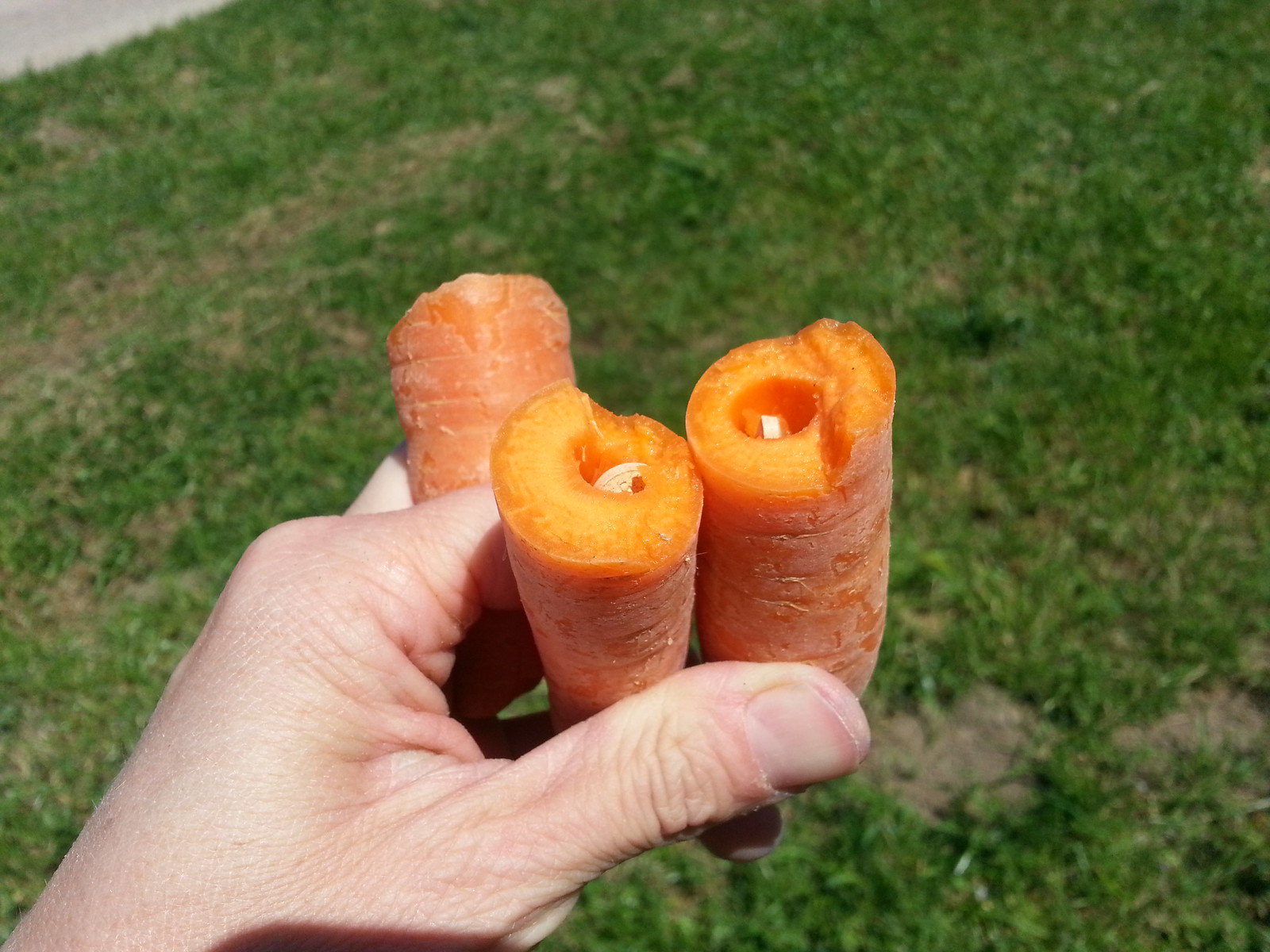A close-up outdoor photograph features the partially visible hand of a pale-skinned individual, likely a young white male. The hand, with neatly trimmed nails, grasps three segments of carrots. Two thick carrot pieces are held between the thumb and forefinger, prominently displaying their interiors, which are hollowed out. Within these recessed cavities, there are curious white structures — possibly the beginnings of roots or some small object, like a bean sprout or white bug. The third carrot segment is clasped between the middle and index fingers, turned slightly to the side.

The carrots appear to be roughly broken rather than neatly cut and remain unpeeled, displaying a slightly aged, whitish exterior. The background focuses on a scruffy, sunlit lawn with visible patches of soil, emphasizing the outdoor setting. The uneven grass appears out of focus, contrasting with the sharp detail of the hand and carrots in the foreground.